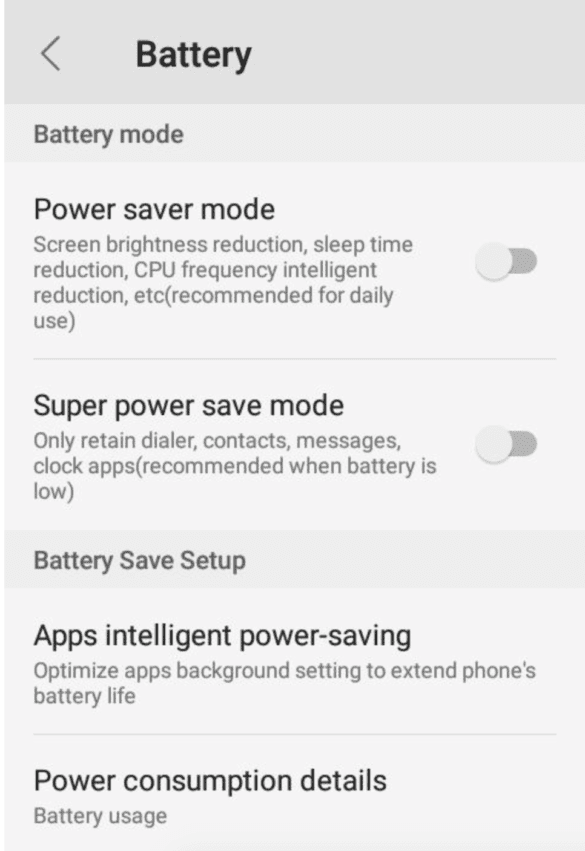The image is a screenshot of an Android phone displaying the battery settings menu, customized with a grayscale color scheme and a standard font. At the top of the screen, a darker gray bar features the word "Battery" in black font with initial capitalization. Directly below, the first subheading area labeled "Battery Mode" appears in a slightly lighter gray and is also in dark gray text.

Under the "Battery Mode" section, two options are listed in black font: "Power Saver Mode," which is turned off, and "Super Power Saver Mode," also turned off. 

Further down, another subsection titled "Battery Save Setup" is presented in a slightly darker gray hue with the title in gray text. In this section, two more items are listed in black font: "Apps Intelligent Power Saving" and "Power Consumption Details." Both of these items are accompanied by more detailed explanations.